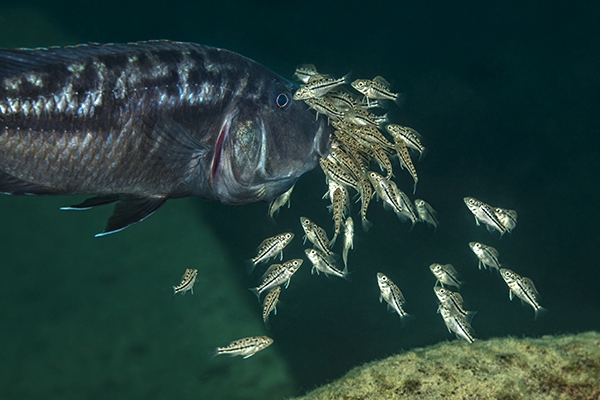This underwater landscape photograph captures a detailed, color-rich scene of a large silver-black fish emerging prominently from the upper left side of the frame. The fish's head is centrally positioned with its tail out of view. It features striking silverish scales, a dark gray face, and a pearlescent pink and greenish gill. Its black eyes are accentuated by a gold ring encircling them. Along its spine stretches a notable fin, while two smaller black fins with white tips project below. Enigmatically, over 20 to 30 small fish — tan, black, gold, and silver, each with tiny black eyes and distinctive stripes or spots — are swarming around its open mouth, creating a dynamic and bustling underwater environment. The background shifts from a dark green hue on the right to a lighter shade on the left, with a cluster of dark green rock or sand on the lower right, enhancing the natural underwater palette.